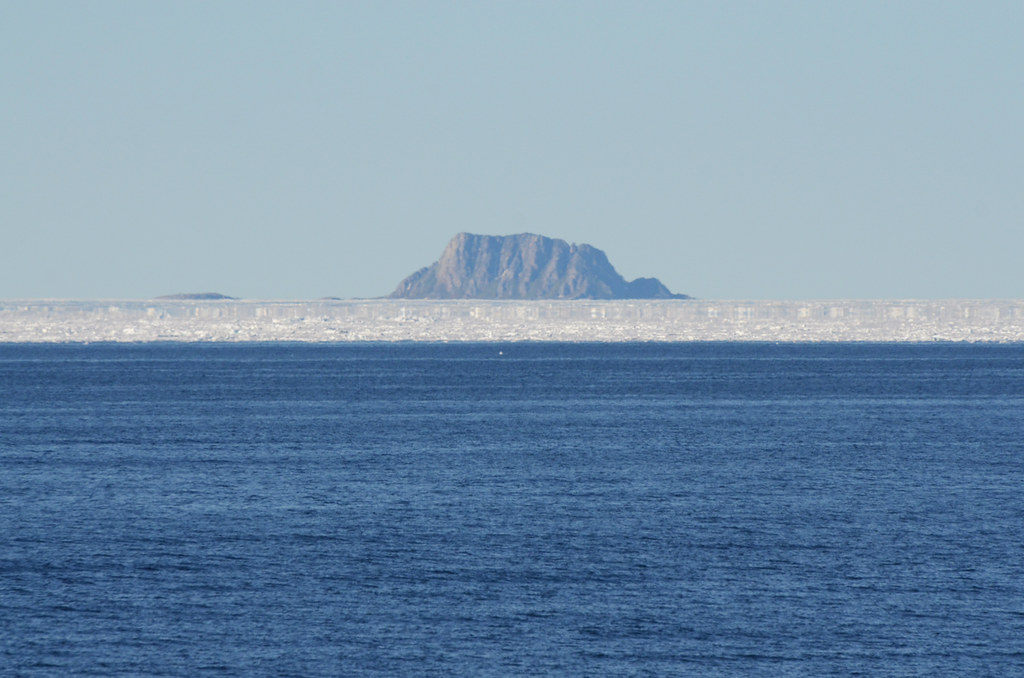The photograph captures the essence of a serene Arctic landscape. The foreground features a vast expanse of dark blue ocean, which extends from the bottom edge of the image up to the middle. The water appears calm, adorned with gentle ripples that create a subtle shimmering effect. In the middle of the photo, a flat, rectangular strip of ice stretches horizontally from left to right, resembling a glacier. This icy band adds a striking contrast to the otherwise smooth ocean surface. Beyond the ice, a rugged, stone mountain rises imposingly in the background, its dark, rocky face standing tall against the horizon. Encircling the mountain is a light grayish-blue sky, seemingly filled with clouds, adding a mystical and serene ambiance to the scene. The sky’s bluish-gray hue seamlessly blends with the distant mountain, completing the peaceful Arctic vista.